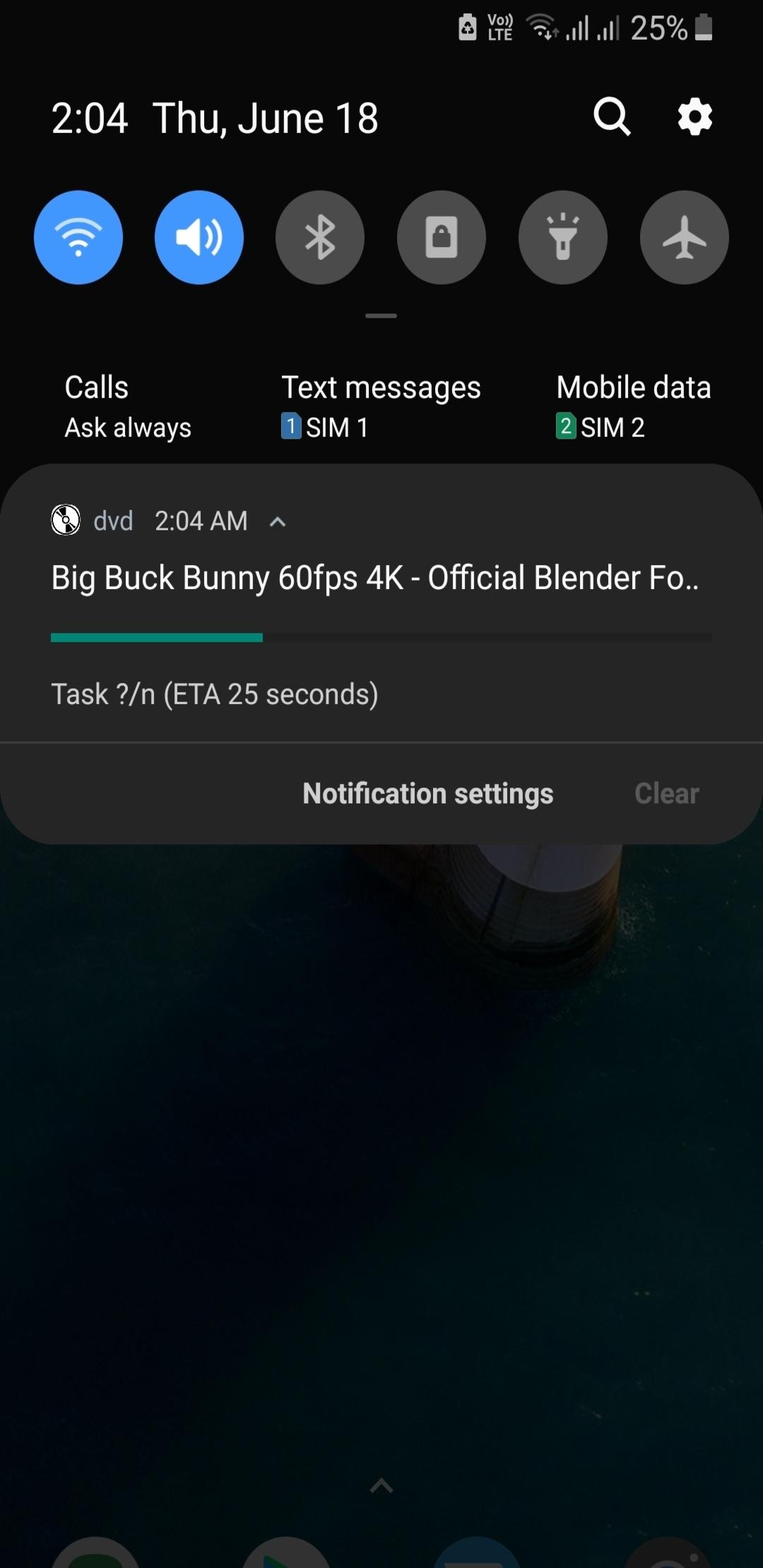This image depicts a screenshot of an Android device's interface. At the top right corner, various status icons are visible, including battery level, cellular signal strength, and Wi-Fi signal. Below these icons, the time is displayed as "2:04 PM" on a Thursday, June 18th. On the far right side of this bar, there are two icons: a magnifying glass for search functionality and a cog representing the settings menu.

Immediately beneath this, a row of circular buttons spans the entire width of the screen. These buttons have different icons; the active buttons are highlighted with a blue background while the inactive ones are greyed out. The active buttons in this screenshot are the Wi-Fi button and the volume button. The other icons represent Bluetooth, a lock symbol, a flashlight, and airplane mode.

Further down, there's a small horizontal line in the center of the screen. Below it, the display is divided into three columns with different settings. The first column says "Calls" with the option "Ask Always," the second column shows "Text Messages" assigned to "SIM 1," and the third column lists "Mobile Data" set to "SIM 2."

A section underneath spans the full width of the screen, featuring a small icon of a disc next to the text "DVD." Beside this, the time "2:04" is shown again, followed by the title "Big Buck Bunny 60fps 4K." Below this title, a progress bar indicates loading at approximately 35%, filled in green. The notification settings option falls beneath this loading bar. The background of the screen features a wallpaper, completing the scene depicted in the screenshot.